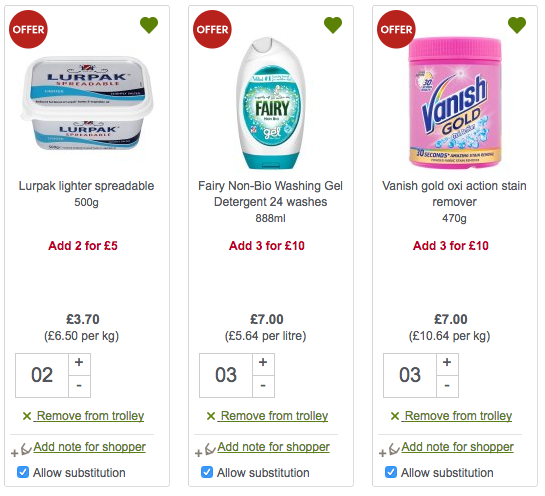**Detailed Caption:**

The image showcases a selection of household items displayed with detailed pricing and purchase options. On the left, there is a white tub of Lerpac Lighter Spreadable, weighing 500 grams. The price is marked at $3.70, with an offer of adding two tubs for five pounds. The cost per kilogram is listed as $6.50. Options to remove it from the trolley, add a note for the shopper, and allow substitution are indicated.

In the center, there is a white bottle of Fairy Non-Bio Washing Gel Detergent, capable of delivering 24 washes. The special offer allows adding three bottles for $10. Individually, each bottle is priced at $7, translating to $5.64 per liter. Similar options to remove it, add a shopper's note, and allow substitutions are provided.

On the right, there is a pink tub of Vanish Gold Oxi Action Stain Remover, priced at $7, which calculates to $10.64 per kilogram. It, too, can be removed from the trolley, have notes added, and substitutions allowed. 

Below each product are symbols for offers, hearts indicating favorites, and checkboxes possibly for selection. Additionally, there are plus and minus signs for adjusting quantities.

This well-organized display clearly delineates the products, making it easier for shoppers to make informed decisions.